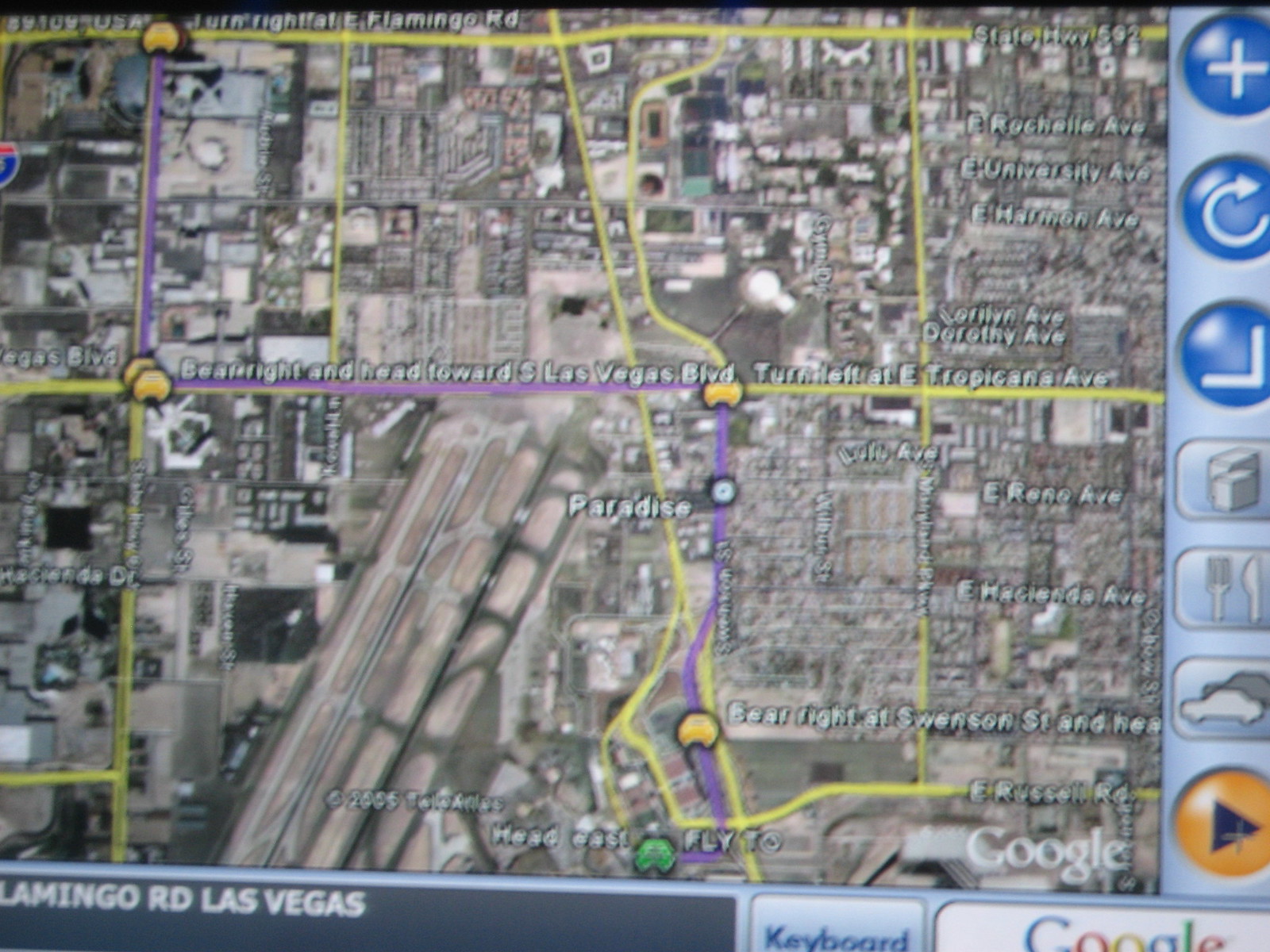The image depicts a navigation screen, likely from a car, displaying a map for directions. On the right side of the screen, vertical blue buttons feature symbols including a plus sign, a rewind icon, an L-shaped arrow, a fork and knife symbol for restaurants, a car icon, and a possible gas tank icon. In the bottom right corner, an orange button with a black triangle appears meant for advancing forward. Beneath the map, text reads "Flamingo RD, Las Vegas," accompanied by a "Keyboard" button and a "Google" logo. The map, featuring a brown and green color scheme with major roads highlighted in yellow or purple, appears blurry and difficult to read. Central on the map are directions stating "bear right and head towards Las Vegas Blvd" above a purple line, with "Paradise" written vertically on a yellow line. Additionally, there's an orange car symbol marked on the map.